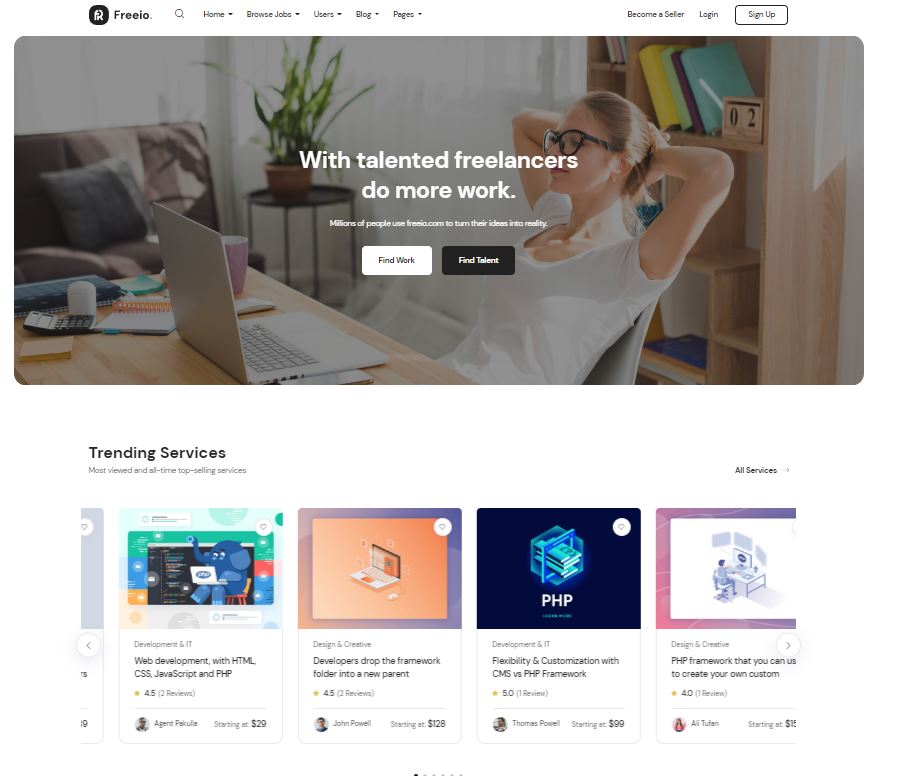Screenshot from the Free.io website. 

The header features the navigation menu with the following options: Home, Browse, Jobs, Users, Blog, and Pages. On the right side of the same row, there are options to "Become a Seller," "Login," and a "Sign Up" button.

The main image showcases an office worker working remotely from home. She is wearing a white T-shirt with "UNIC" printed on it. She has black-rimmed glasses and is sitting in front of a table with an open laptop. Her hands are comfortably placed behind her head. Below the image, a text reads, "With talent, freelancers do more work." 

Two buttons are positioned toward the bottom of the image: a white button labeled "Find Work" and a black button labeled "Find Talent" in white text.

Underneath this section, there is a "Trending Services" section on the left side containing four service categories:
1. **Web Development:**
   - Technologies: HTML, CSS, JavaScript, PHP
   - Starting at $20
   - Rating: 4.5 stars

2. **Framework Implementation:**
   - Service Description: Developers drop the framework folder into a new parent
   - Starting at $128
   - Rating: 4.5 stars

3. **Flexibility and Customization:**
   - Technologies: CMS via PHP framework
   - Starting at $99
   - Rating: 5 stars

4. **Custom Design Creation:**
   - Technology: PHP framework
   - Starting at $100
   - Rating: 4 stars